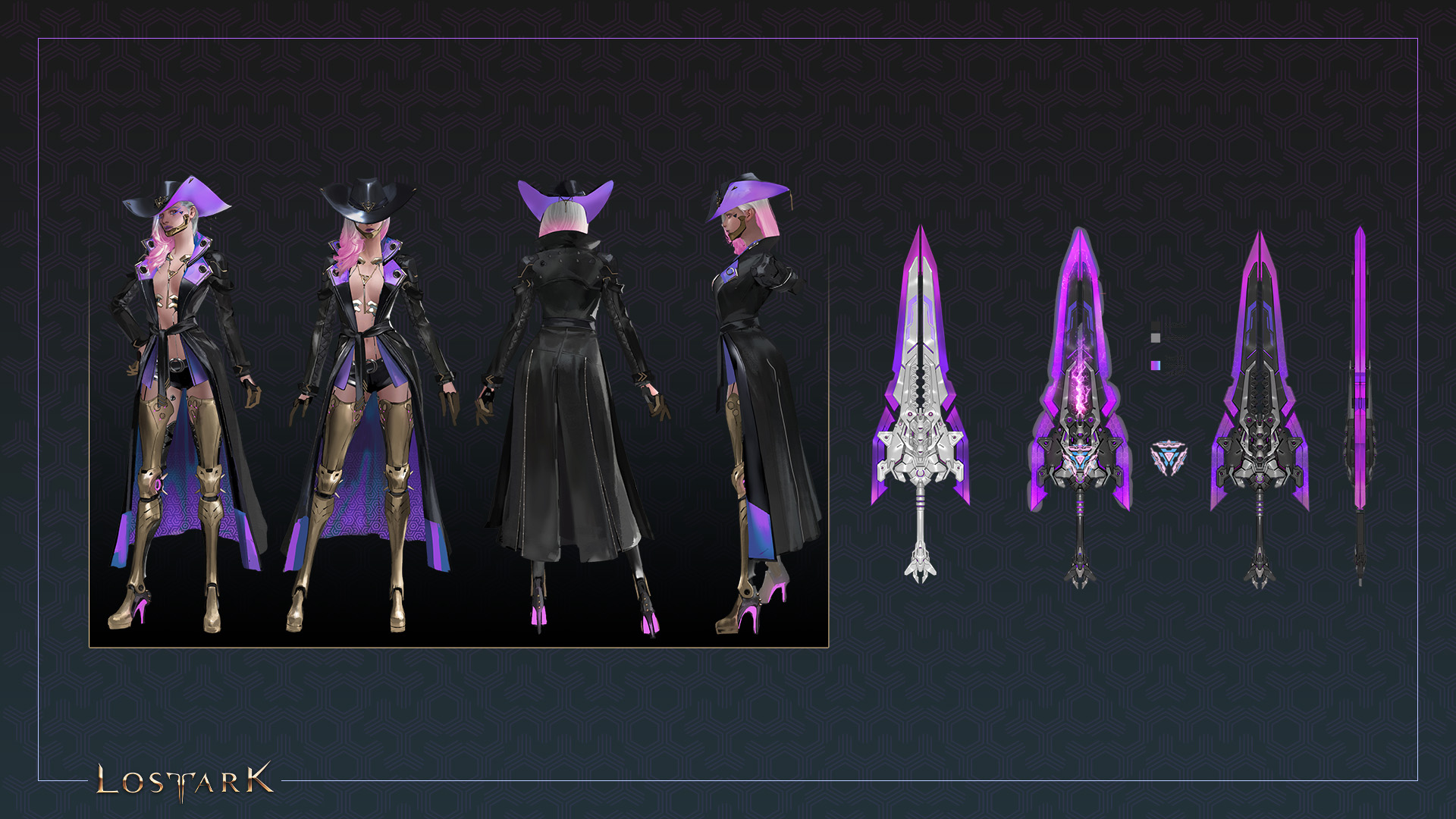The illustration titled "Lost Ark" features a dark slate gray background with a thin, pale gray margin inset about an inch from the edge. The central image is adorned in striking neon purple and blue highlights. The left side showcases four detailed views of a robotic woman with blonde hair and a commanding presence. She wears a large floppy black hat with a purple underside, and a long black trench coat, the inside of which is illuminated with the same purple and blue hues. Under the coat, she sports a bikini-like outfit and high-heeled shoes or boots, the undersides glowing with a pinkish hue. The views include her front, a front view looking down showcasing the top of her hat, a rear view revealing her belt and the inside of her coat, and a left profile.

To the right, four depictions of a sci-fi, futuristic sword or weapon complement the image. Each blade is rendered in gray with neon purple and blue highlights, portraying the weapon from different angles — front, rear, and side. The word "Lost Ark" is prominently displayed at the bottom left of the illustration. This intricate and vividly colored artwork portrays a strong, robotic heroine in various detailed poses, alongside her weaponry, emphasizing a fusion of futuristic and fantastical elements.